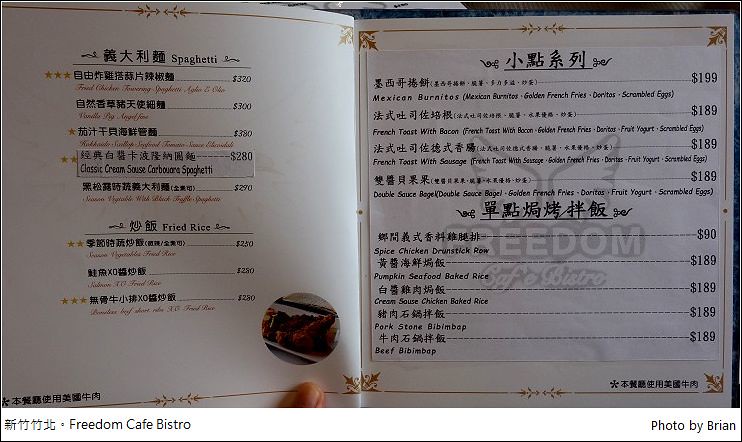This screenshot captures the menu of the Freedom Cafe Bistro, with the name prominently displayed in black lettering in the lower-left corner. To the right of the name, the photo is credited to Brian. The menu has an intriguing blend of cuisines, primarily showcasing American dishes, yet it closely resembles the format of a Chinese menu. It is presented on a white background with what appears to be paper taped over some sections. 

A distinctive yellow border frames the menu pages, and at the corners, there are orange-yellow fleur-de-lis-like logos adding a touch of elegance. Despite some of the text being in Chinese or Japanese, several dishes are clearly listed in English. The menu items include a variety of international flavors such as Classic Cream Carbonara Spaghetti, Mexican Burritos, French Toast with Bacon, French Toast with Sausage, Double Sauce Bagel, Spiced Chicken Drumstick Roe, Pumpkin, Seafood Baked Rice with Cream Sauce, Chicken Baked Rice, Pork Stone Bibimbap, and Beef Bibimbap.